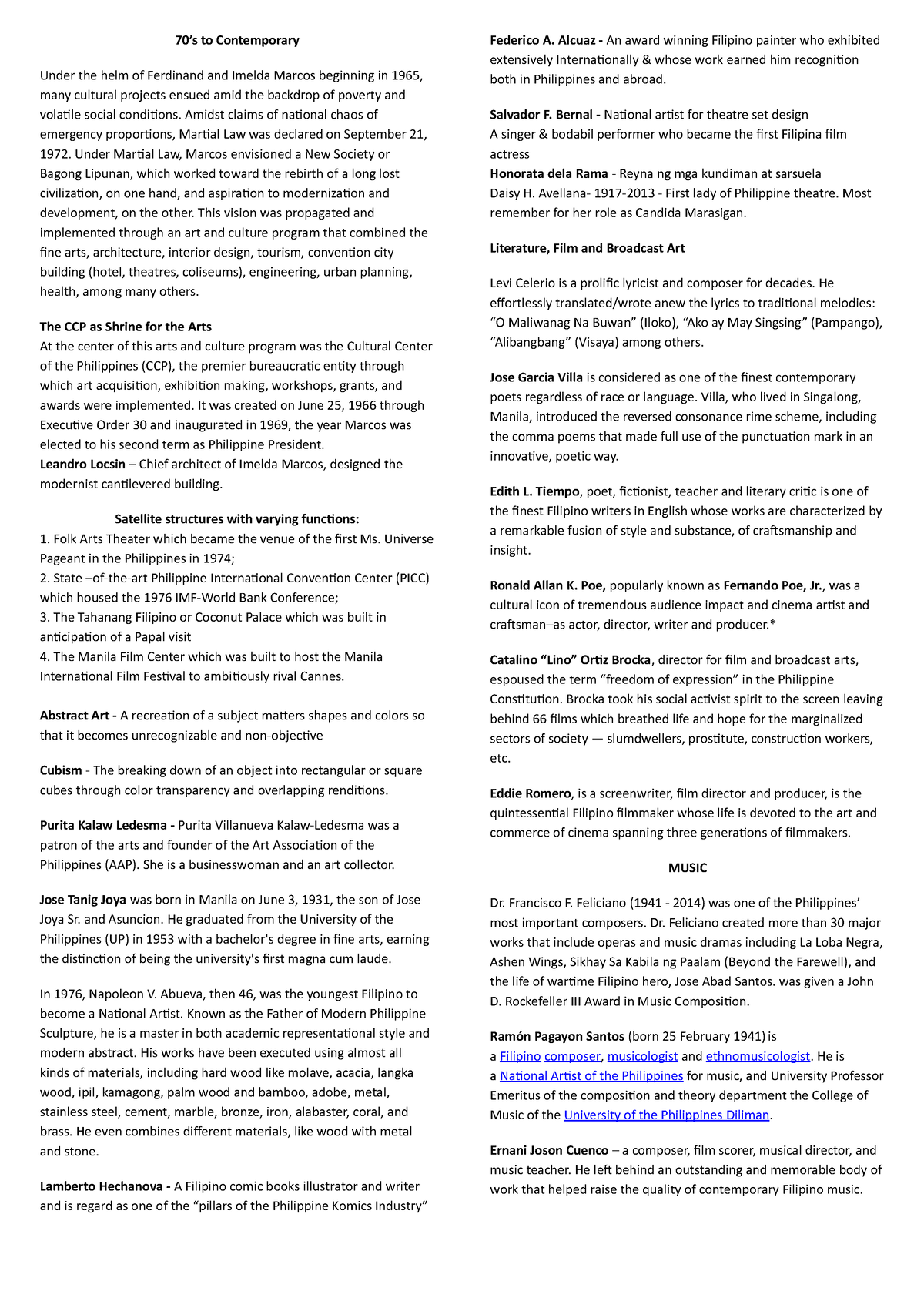This is an image taken from a device screen, displaying a detailed historical text titled "70s to Contemporary." The text delves into the cultural and political landscape of the Philippines under the rule of Ferdinand and Imelda Marcos, starting in 1965. It highlights how numerous cultural projects were initiated against a backdrop of poverty and volatile social conditions. The narrative notes the declaration of martial law on September 21, 1972, amidst claims of a national emergency. Under martial law, Marcos pursued his vision of a "New Society" or "Bagong Lipunan," aiming for the rebirth of a long-lost civilization. This vision sought modernization and development and was promoted through an arts and cultural program encompassing fine arts, architecture, interior design, tourism, and more.

The text further includes a section titled "CCP as Shrine for the Arts," elaborating on various aspects like satellite structures with diverse functions, abstract art, and cubism. It covers multiple forms of artistic expression, including music, literature, film, and broadcast art, presented in two detailed columns. At the bottom of the screen, there are clickable links in blue for additional information.